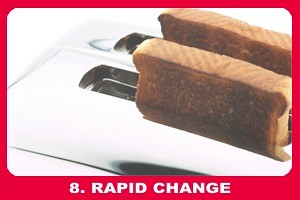The image features a close-up of a bright, silver two-slot toaster with two pieces of toast that have just popped up. The toast appears to be well-done, with dark brown toast marks clearly visible against the tan tops. The toaster sits at an angle, allowing a detailed view of both pieces of bread, including the top crusts. The photo is presented within a red digital frame, making the white background and the shiny toaster blend slightly, creating a dazzling effect. At the bottom of the red border, white text reads "8. RAPID CHANGE," indicating the image's title or position in a sequence.